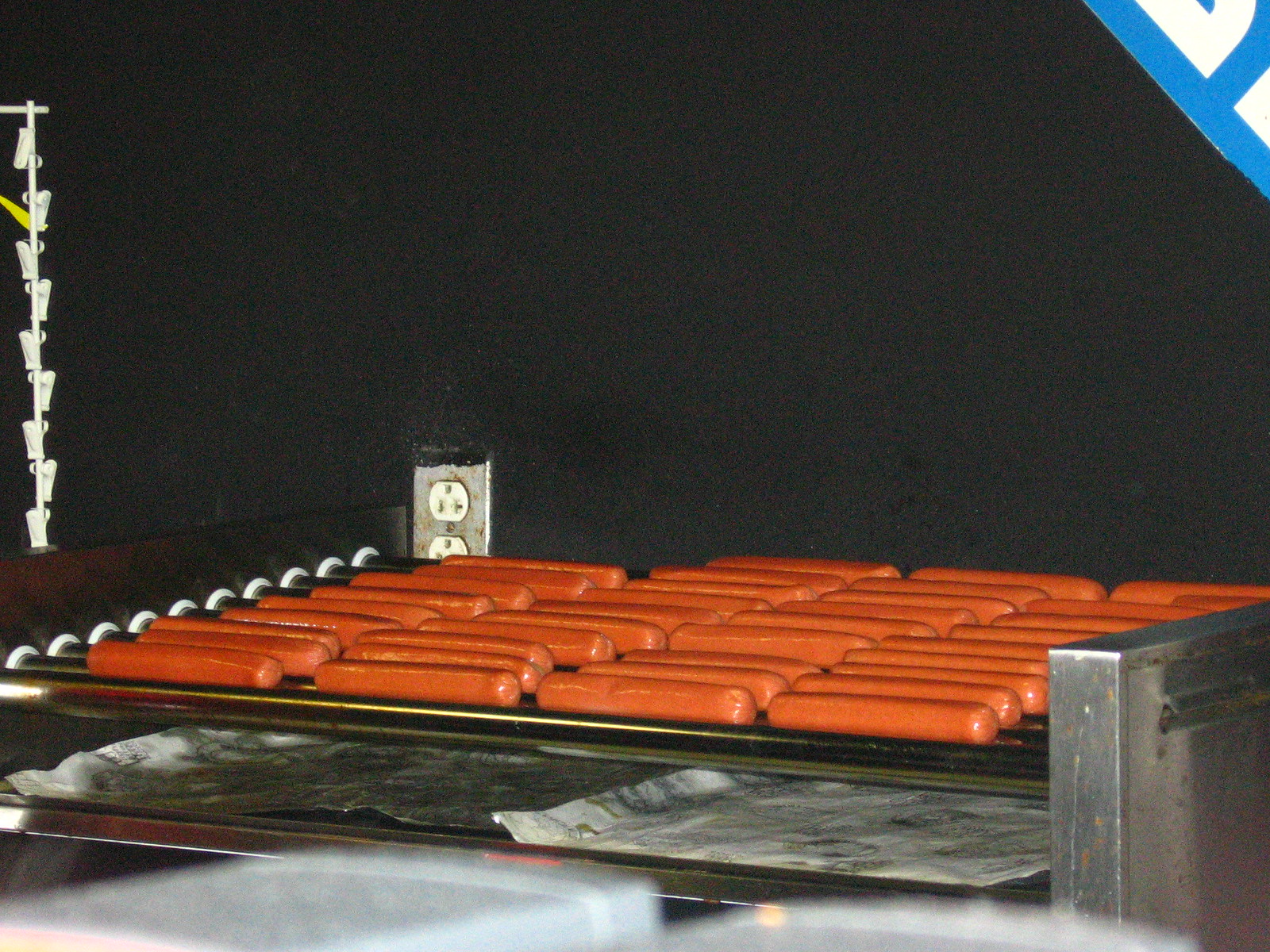The image depicts a horizontal, rectangular photograph of approximately four dozen hot dogs cooking on a stainless steel electric rotisserie grill, commonly found in convenience stores. The hot dogs are arranged in four horizontal rows on the rotating rollers, which spin them evenly. Below the hot dogs, a drip pan is visible. The stainless steel grill features silver sides and rollers, which are attached to the frame with white circular washers. In the background, the wall is black, and slightly left of the center is a stainless steel electrical outlet with a three-way plug and some black paint and rust on its surface. A distinctive blue and white square is present in the upper right-hand corner of the image. On the left side, a rod with metal clips, typically used for holding small bags of chips, hangs down, and a piece of yellow bag hangs from one of the clips. The entire background is predominantly black, emphasizing the cleanliness and metallic sheen of the hot dog grill.